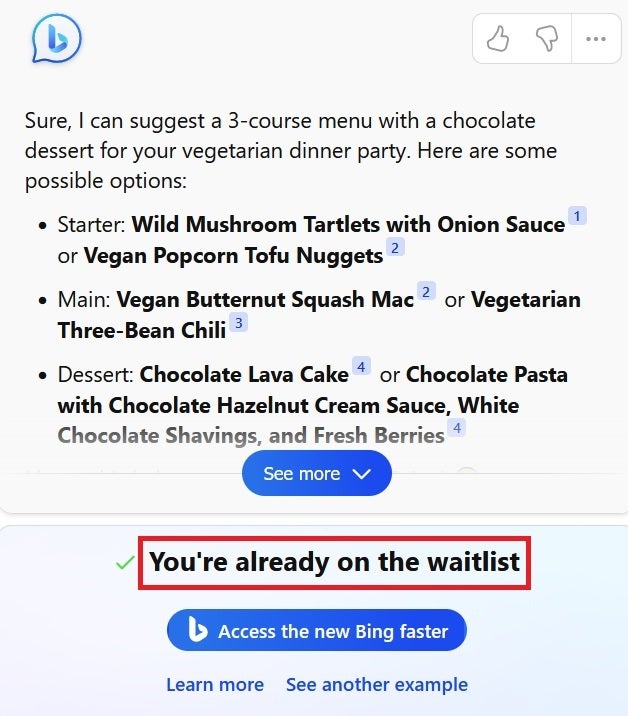Screenshot of a dialogue box displaying a suggested 3-course menu for a vegetarian dinner party. The header reads, "Sure, I can suggest a 3-course menu with a chocolate dessert for your vegetarian dinner party. Here are some possible options."

The menu is organized as follows:

**Starter:**
- **Wild Mushroom Tartlets with Onion Sauce**
- **Vegan Popcorn Tofu Nuggets**

**Main:**
- **Vegan Butternut Squash Mac**
- **Vegetarian Three Bean Chili**

**Dessert:**
- **Chocolate or Chocolate Pasta with Chocolate Hazelnut Cream Sauce, White Chocolate Shavings, and Fresh Berries**

Below the menu options, there's a button labeled "See More." Underneath that button, a message reads, "You're Already on the Waitlist," followed by a prompt, "Access the new Bing faster."